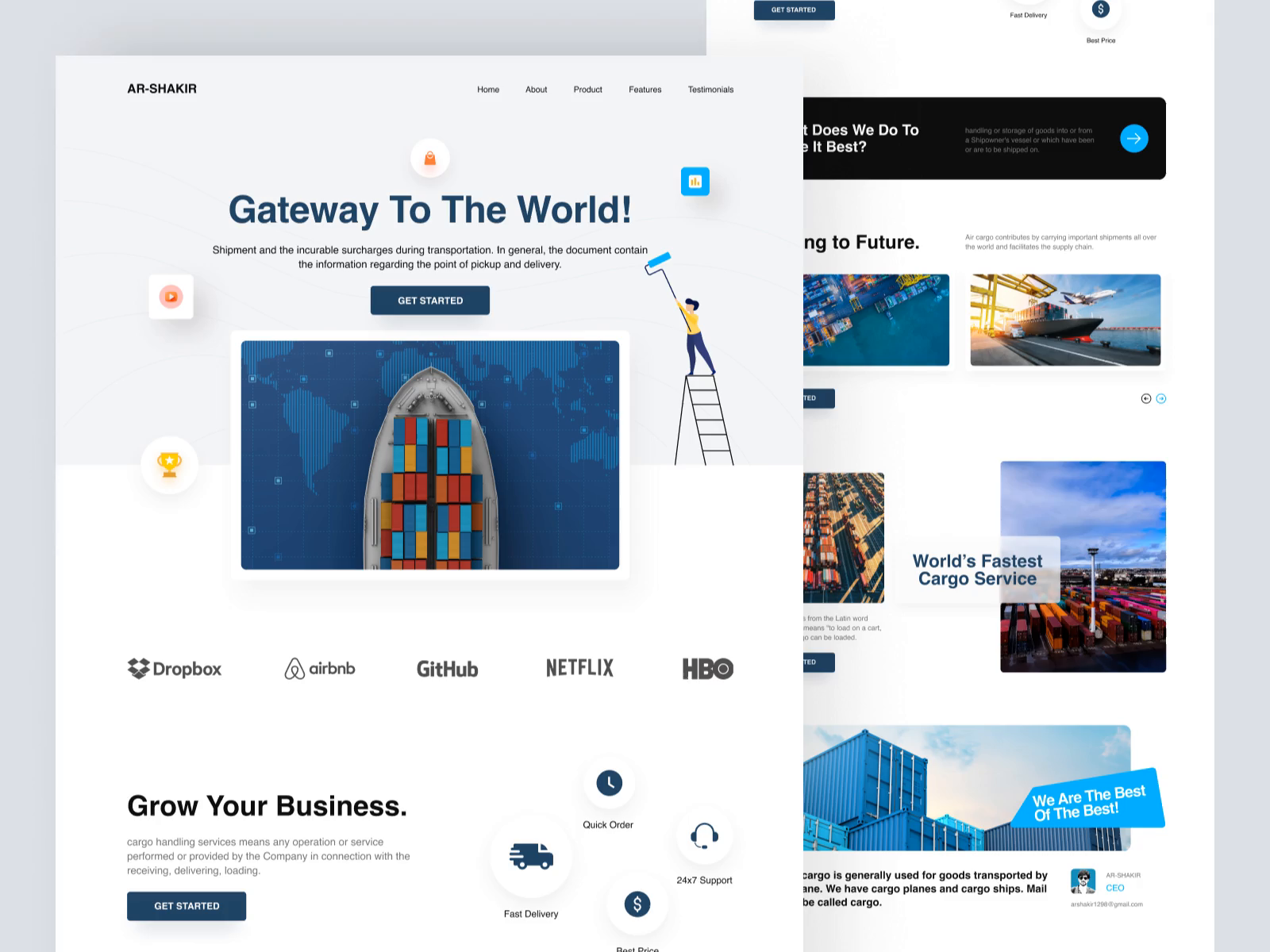A screenshot of a website featuring a predominantly white background with a light gray vertical border along the right side and a gray vertical column on the left that extends upward and intersects with the middle. The top-right corner showcases a dark blue "Get Started" button. Above this button, black text reads "Fast Delivery," accompanied by a blue circle with a dollar sign and the text "Best Price."

In the top-left corner, within the white area, the name "AR-Shakir" is displayed, and to its right are five navigation options in black text: "Home," "About," "Product," "Features," and "Testimonials." Centrally positioned at the top is a white circle with an orange lock, surrounded by the prominent blue text "Gateway to the World." Below this, smaller black text states, "Shipment incurable surcharges during transportation."

In the middle section of the website is an image of a container ship viewed from above, loaded with various colored containers, superimposed on a blue map of the world. Directly below this image are logos of well-known companies: Dropbox, Airbnb, GitHub, Netflix, and HBO. Beneath the logos, four buttons labeled "Fast Delivery," "Quick Order," "24/7 Support," and "Best Price" are aligned horizontally.

At the bottom left, black text reads, "Grow Your Business. Cargo handling service means any operation or service performed or provided by the company in connection with receiving, delivering, loading." Another dark blue "Get Started" button is located at the bottom center of the page.